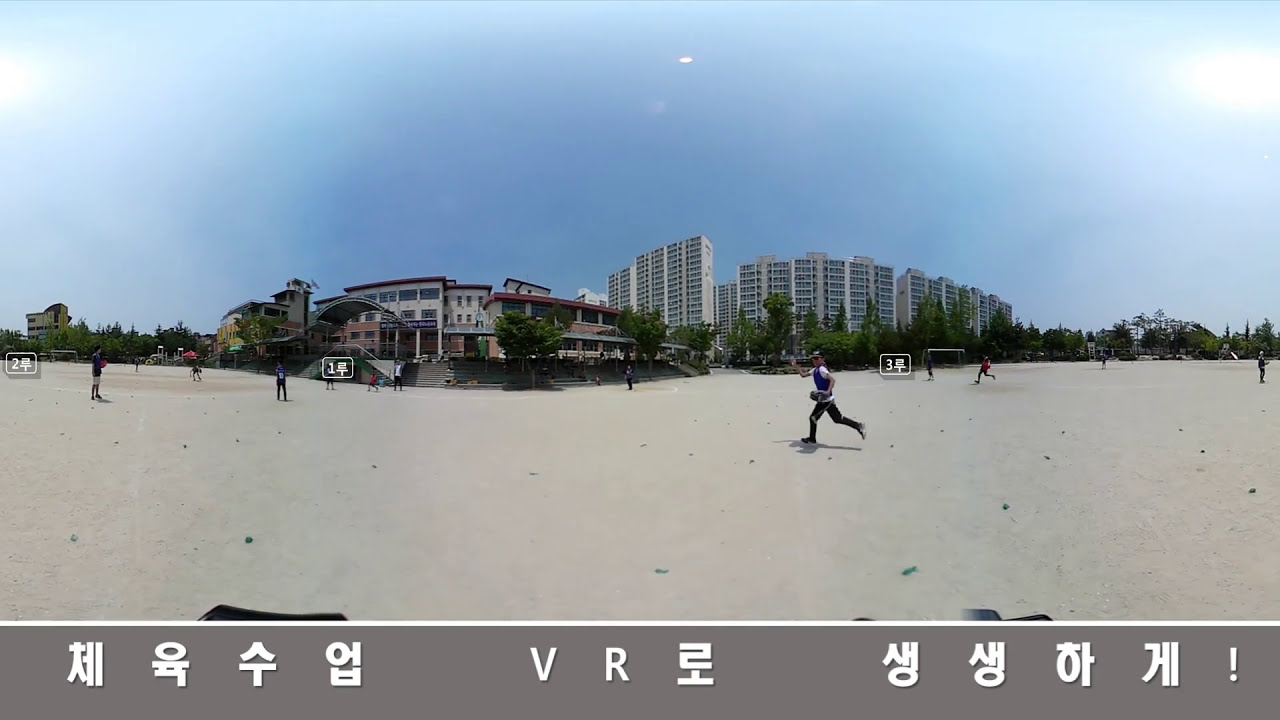The image showcases a bustling beach scene during a sunny day with a clear blue sky. At the forefront, several people are actively running on the sand, seemingly engaged in a game of baseball. The vibrant panorama also features other beachgoers walking leisurely along the shore. A distinct Photoshopped effect is apparent, creating an unusual visual element with two Suns visible on either side of the picture.

In the background, tall skyscrapers and shorter buildings, possibly hotels and stadium-like structures, line the beach, contributing to a cityscape vibe. The entire scene is enriched with lush trees adding to the natural beauty. 

Overlaying the image, white-outlined numbers with Asian characters are scattered - a "2" on the left, a "1" near the stadium-like building, and a "3" by the skyscrapers, indicating a sequenced or augmented reality element. At the bottom, a gray footer contains Asian text, interspersed with the letters "VR" and punctuation marks.

The combination of vivid colors, dynamic activity, and intricate layers of text and imagery suggests a complex, manipulated photo that merges reality with digital enhancements.